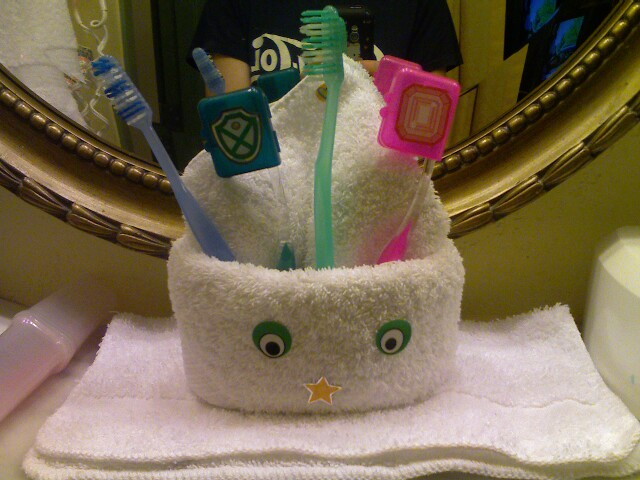This image depicts an up-close view of a whimsical, cartoon-like towel animal in a bathroom setting, fashioned to serve as a toothbrush holder. The towel animal, resembling a child's beanie hat, is crafted from a white, fluffy towel and features two green-bordered googly eyes and a yellow star for a nose or mouth. The creature is perched on another folded white towel, enhancing its playful design.

The towel animal holds four toothbrushes in a pocket formed by its cuffed "head": a blue toothbrush on the left, a green toothbrush next to it, another green toothbrush with a clear handle and a cover on its brush head near the center, and a pink toothbrush with a protective cap on the right. Next to the towel animal, there is an empty pink and clear toothbrush case.

In the background, a large, round mirror with a gold frame hangs on the wall, partially reflecting a person in a black t-shirt holding a phone to take the photograph. On the right side of the image, the edge of a sink is visible, indicating the bathroom setting.